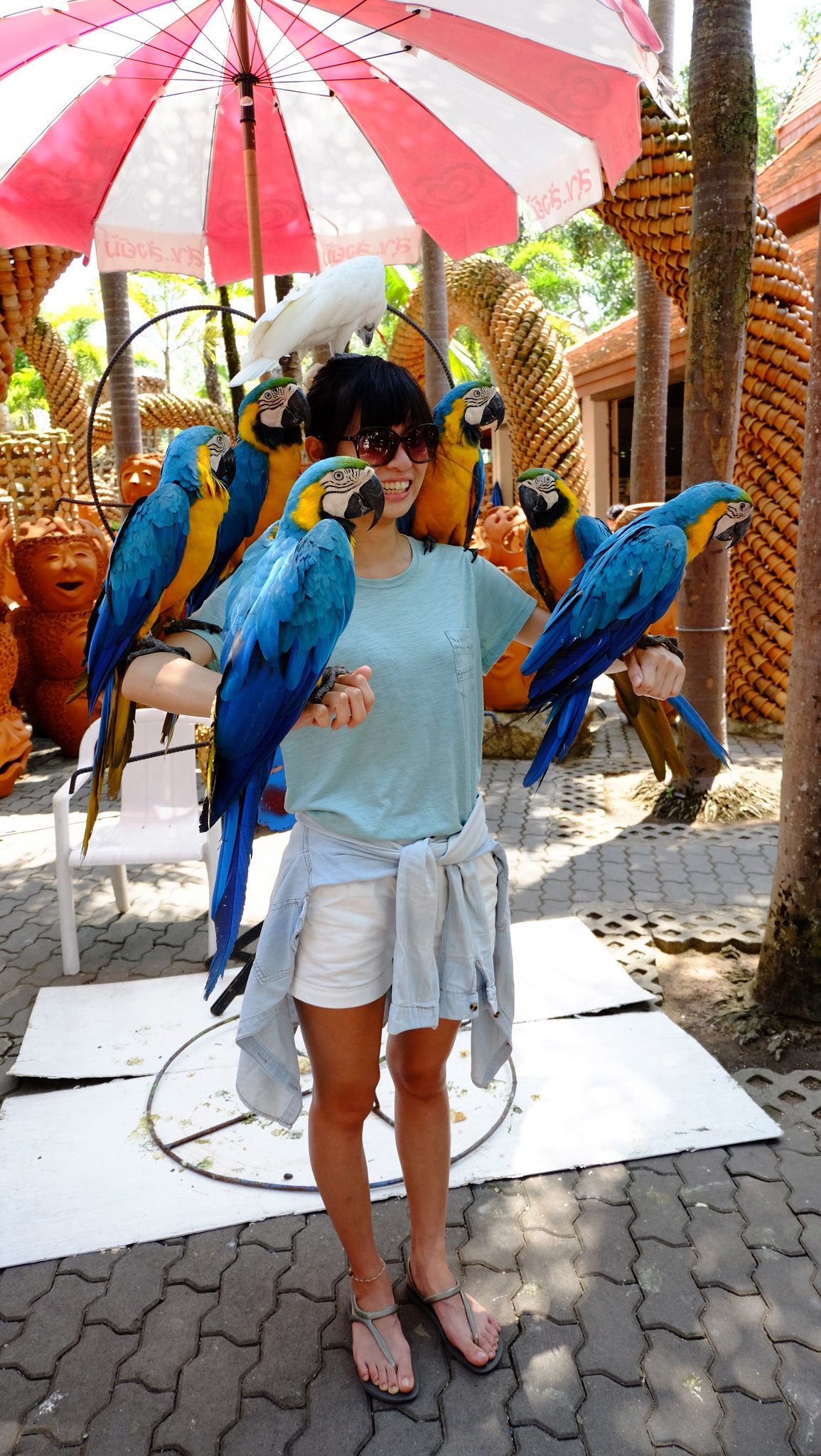In the image, a girl with short black hair is standing in the center on a grey concrete surface, surrounded by a vivid display of colorful birds. She is wearing big black sunglasses, a light blue short-sleeved shirt, white shorts, and a light grey jacket tied around her waist, along with sandals. Her arms are outstretched and bent at the elbows, with her fists closed and knuckles facing the camera. Perched ornately on her arms, shoulders, and head are a total of six birds.

On her left arm, right at the elbow, sits a parakeet with a blue back, yellow stomach, and big black beak. On the front of her right wrist is another parakeet, featuring a blue back, red jaw, white face, and black beak. Behind her, resting on her shoulders, are two more birds, each with a yellow chest, blue head, and black beak.

On top of her head stands a white bird, which is looking away from the camera. On her right elbow, closest to the camera, is a parakeet with a yellow belly, blue wings, white face, and black beak. Lastly, on her left wrist is a parakeet with a blue head and back, purplish feathers, yellow behind its eyes, white face, and black beak.

The background features beach-themed decorations, including wicker baskets and a prominent pink and white umbrella, enhancing the vibrant and lively atmosphere of the scene. The cobbled stone area and the outdoor setting suggest a bright, pleasant day, contributing to the image's cheerful and colorful dynamics.